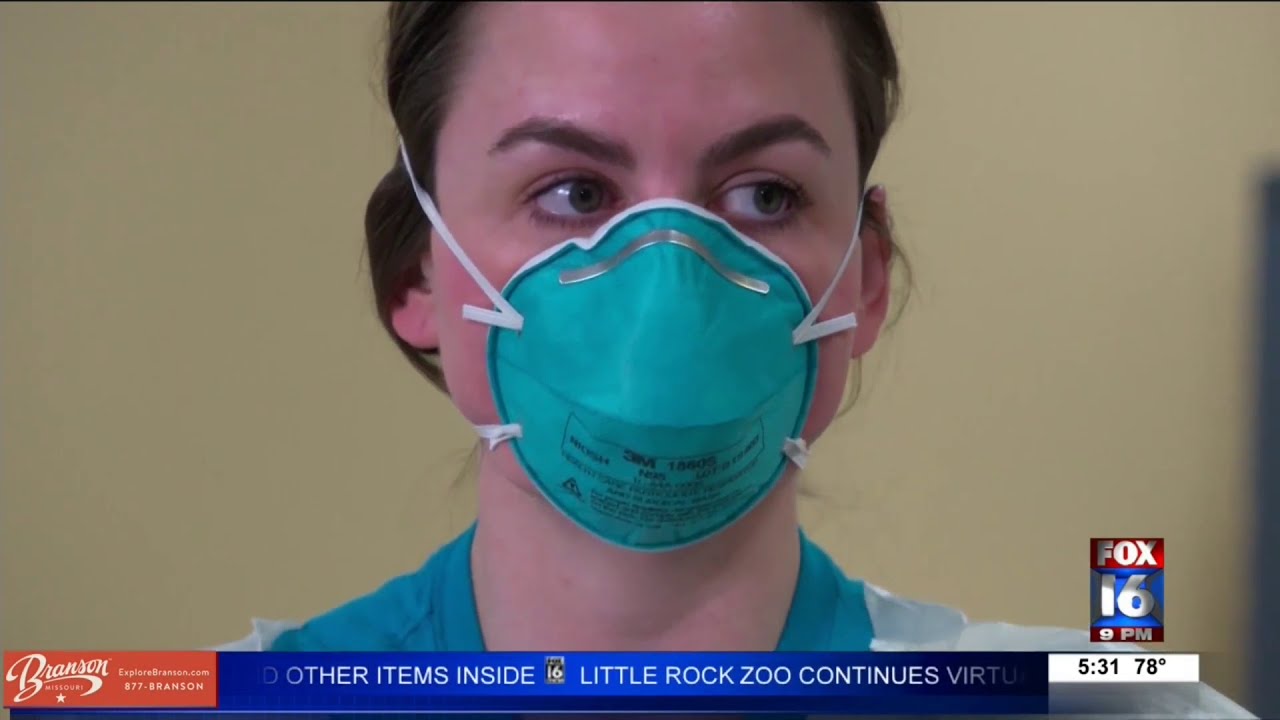The image is a screen capture from a Fox 16 news broadcast, featuring a close-up of a nurse from the shoulders up. She is dressed in a blue shirt under a white lab coat, with a green N95 mask securely fitted over her face, fastened with latex bands. The nurse, who appears to be in her late 30s, has brown hair tied back, thick brown eyebrows, and green eyes. She is looking off to the side, likely being interviewed. 

At the bottom of the screen, a scrolling news ticker reports local news, partially reading, "other items inside. Little Rock Zoo continues virtual..." The time displayed is 5:31 PM with a temperature of 78 degrees. On the bottom left corner, there's a corporate sponsorship logo in white lettering on an orange background, partially reading "Branson." The top part of the screen shows the Fox 16 logo, indicating the news at 8 PM.